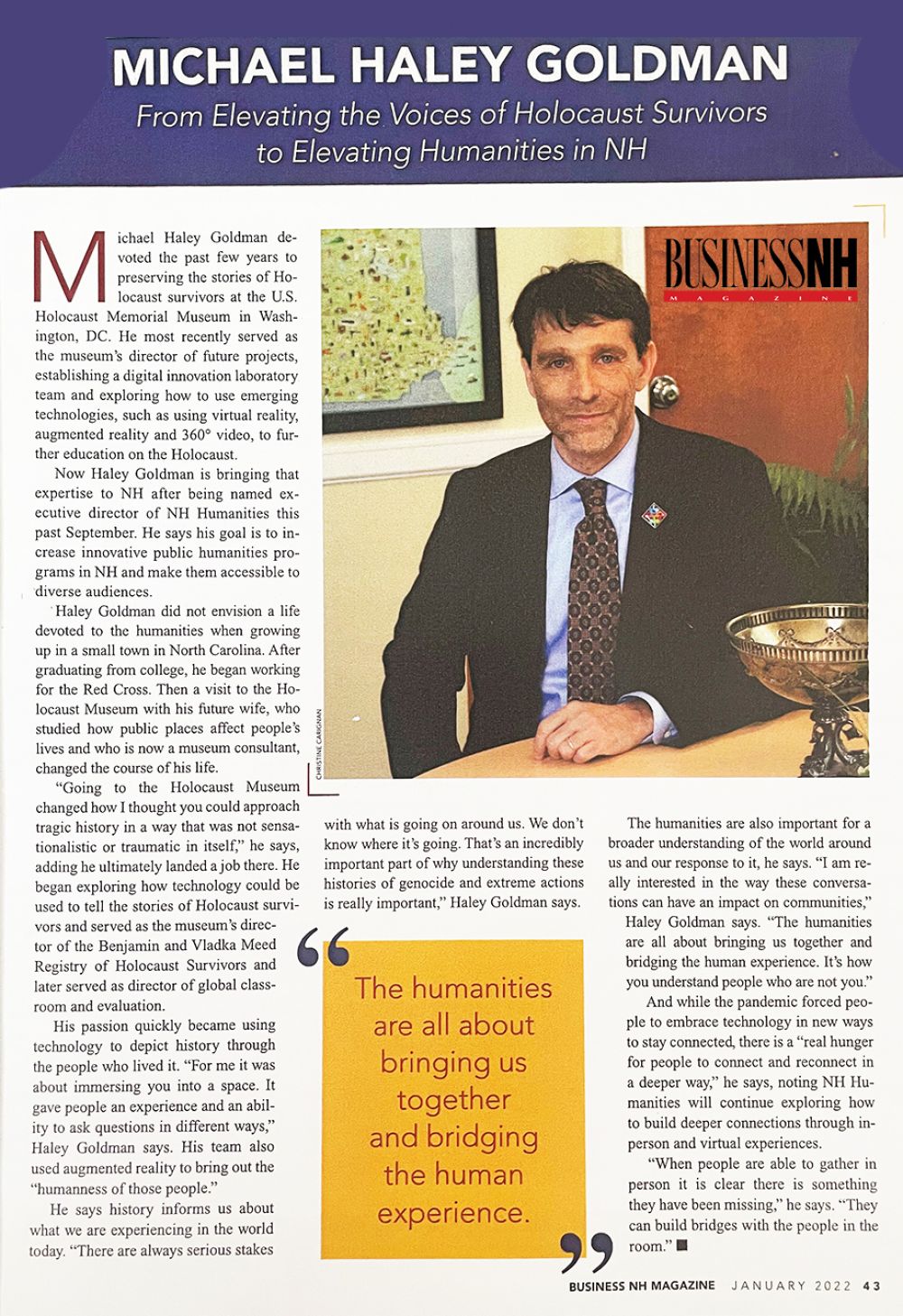This image is a scanned article from the January 2022 issue of Business NH Magazine, found on page 43. The article is titled "Michael Haley Goldman: From Elevating the Voices of Holocaust Survivors to Elevating Humanities in New Hampshire," and it's presented in white text on a purple background. The article features a photograph of Michael Haley Goldman, who is seated at a table, smiling at the camera while dressed in a suit jacket and tie. Overlaid on the photo is Business NH Magazine's watermark, written in black font with "magazine" in white font on a red background below it. A highlighted quote from the article reads, "The humanities are all about bringing us together and reaching the human experience." The piece discusses Goldman's efforts in honoring Holocaust survivors, emphasizing the importance of remembering their stories and combating hatred towards Jews and other minorities in contemporary society.